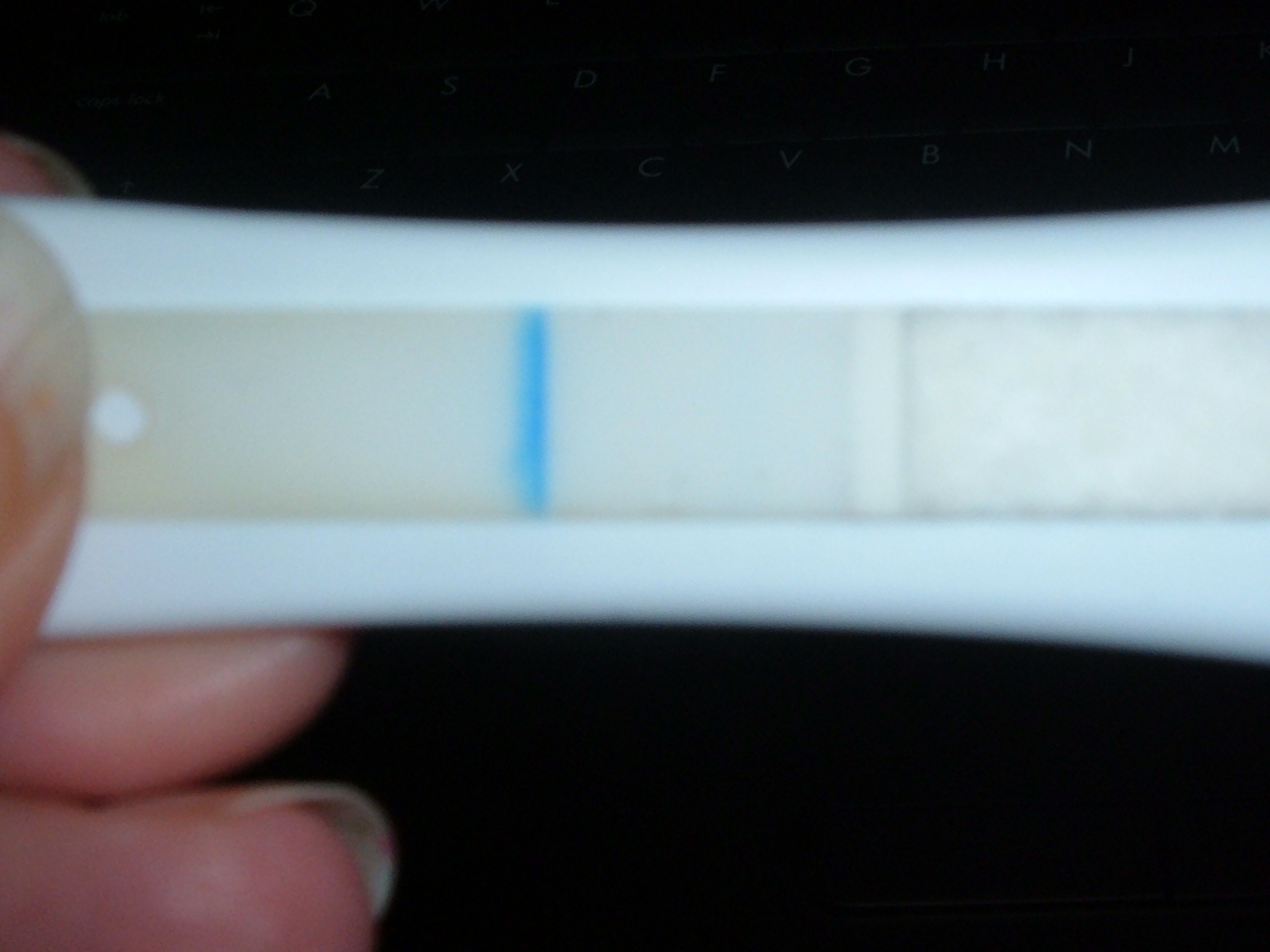The image features a stark, pitch-black background devoid of any identifiable elements. Dominating the foreground, a hand partially appears, revealing the tip of a thumb, a portion of a thumbnail, and a couple of fingers. These fingers are delicately holding a small, white rectangular object. The device, though undeniably a test of some kind, lacks distinguishing marks or clear indicators of its purpose. Positioned towards the left of the white rectangle is a small, white dot. In the center of the rectangle, there's a single, light teal-blue line running horizontally. Despite its evident function as a test, it is not reminiscent of common tests like those for COVID-19, pregnancy, or insulin levels. The test remains an enigmatic object, its true purpose undetermined from the details provided in the image.